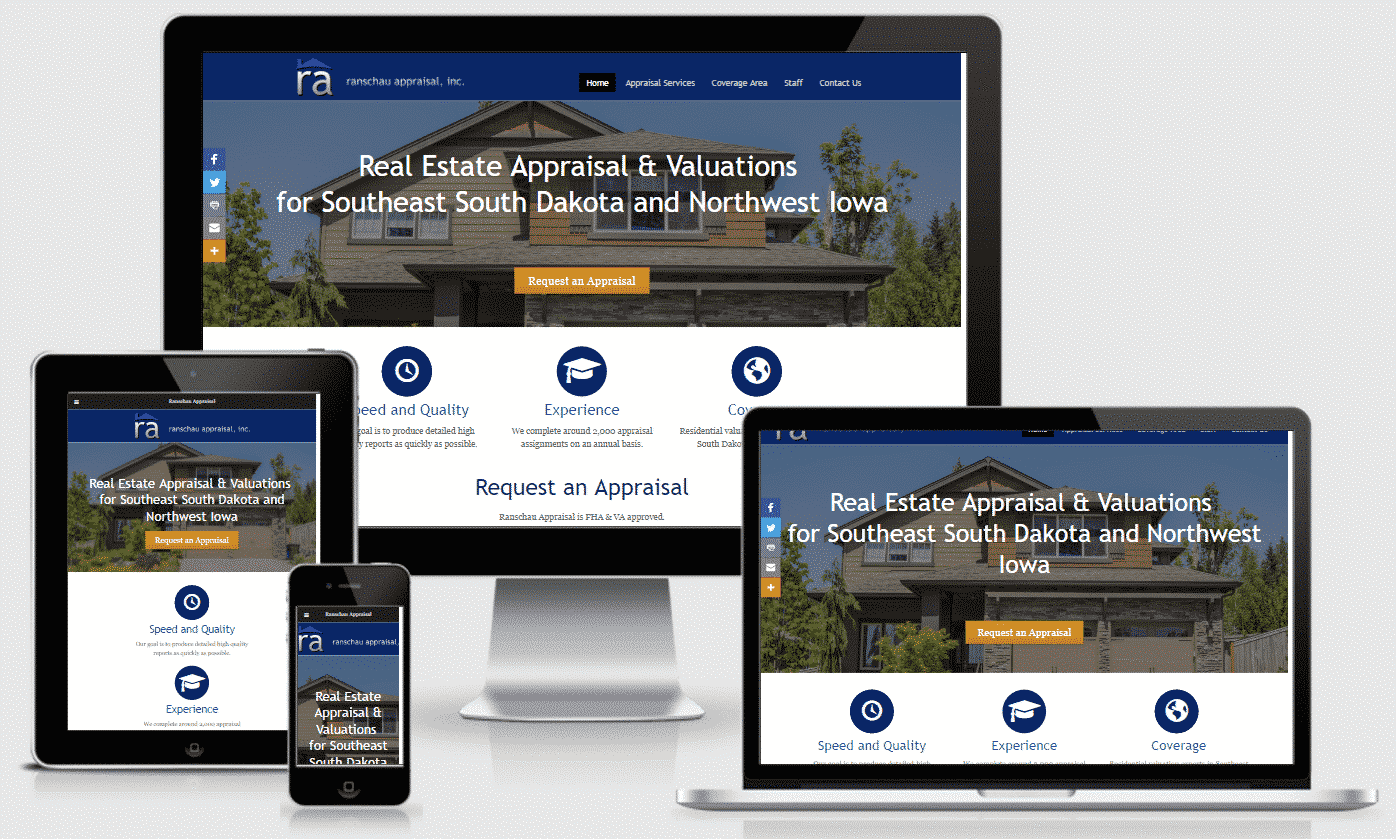This image depicts a design mock-up showcasing a responsive website for a real estate appraisal service, presented across various Apple devices. On the left, an iPad and an iPhone display the homepage, while on the right, a MacBook Pro features the same website. Central to the arrangement is an Apple monitor with a silver base, also exhibiting the website's layout.

The website prominently reads "RA Real Estate Appraisal," specializing in property valuations for Southeast South Dakota and Northwest Iowa. A large hero image of a house serves as the background, enhancing the site’s visual appeal. Below the hero image, three circular icons signify key service aspects: a clock for speed, a graduate cap for quality and experience, and a globe for coverage. Each device casts a realistic, faux reflective shine on the surface below, adding to the mock-up's polished look.

The backdrop is a gradient grey screen, but the overall image quality appears grainy. Nevertheless, the website itself presents a clean and professional design, featuring social media icons for Facebook and Twitter on the left. A call-to-action button, though unclear in text, presumably invites users to request a report or appraisal. This mock-up efficiently demonstrates how the website will appear across multiple devices, ensuring a uniform and accessible user experience.